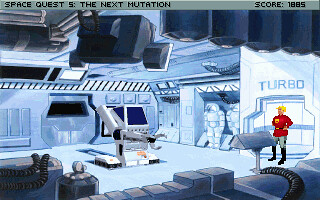The image depicts a scene from the computer game "Space Quest 5: The Next Mutation." At the top of the image, the title is prominently displayed, alongside a score of 1885. The scene appears to be set in a spaceship or a control room, rendered in various shades of blue, from deep navy to light cyan, creating a futuristic ambiance.

Centrally positioned in the image is a character with blonde hair, dressed in a distinctive red short jacket, grey pants, and black boots. The character is engaged with a freestanding console, suggesting they are in the midst of operating or monitoring something important. Behind the character, a doorway marked "Turbo" is visible, adding to the high-tech setting of the space environment.